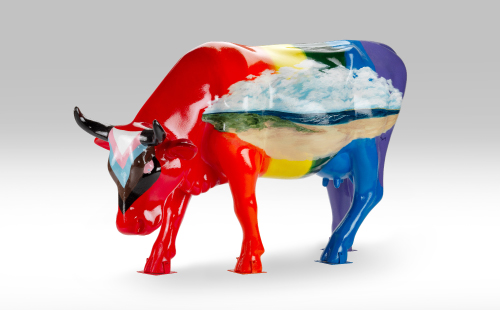The image is a detailed 3D computer rendering of a multicolored cow resembling a rainbow. It features a side view with the cow facing left. The cow's horns are black. The background gradient is gray at the top, transitioning to white at the bottom. Intricately embedded within the cow's body is a picturesque landscape scene. This scene showcases a sky filled with white, fluffy clouds above, a blue ocean with gentle waves, and a strip of green land on the left side. The overall rendering creates a surreal and vibrant juxtaposition of natural elements within the cow's form.